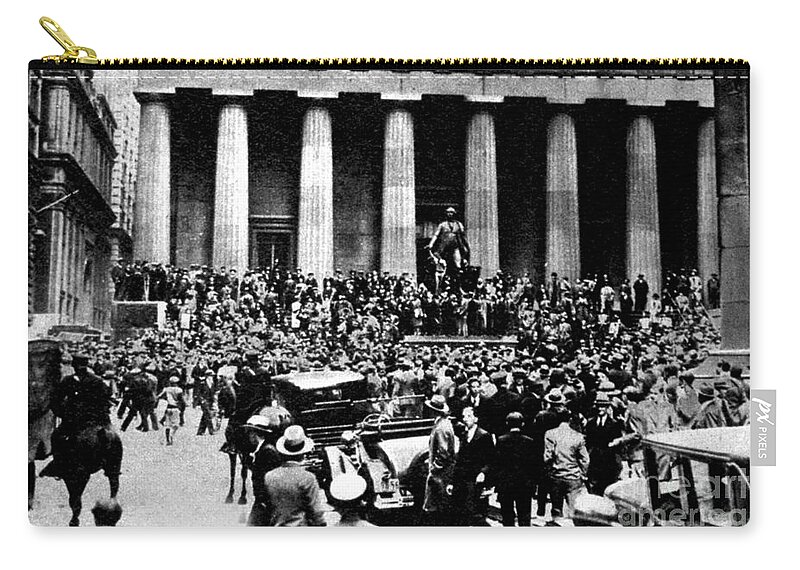This image, imprinted on what appears to be a small, flat, rectangular coin purse with a golden zipper at the top, showcases a detailed black and white photograph. The focal point of the photograph is a large crowd predominantly consisting of well-dressed men in suits and hats, suggesting an era from the 1940s or 1950s. The men are gathered in front of a grand building that resembles a government or monumental structure, characterized by its heavy, ancient Greece-like columns—specifically eight large pillars. These columns frame a doorway behind a prominent statue situated at the center of the scene. Additional details, such as old cars similar to Model T Fords and people on horses, enhance the historical ambiance. The crowd is denser near the statue and building's entrance, with fewer people toward the back. The lower right corner of the purse features a light gray tag with the white text "pixels" and the initials "PX."